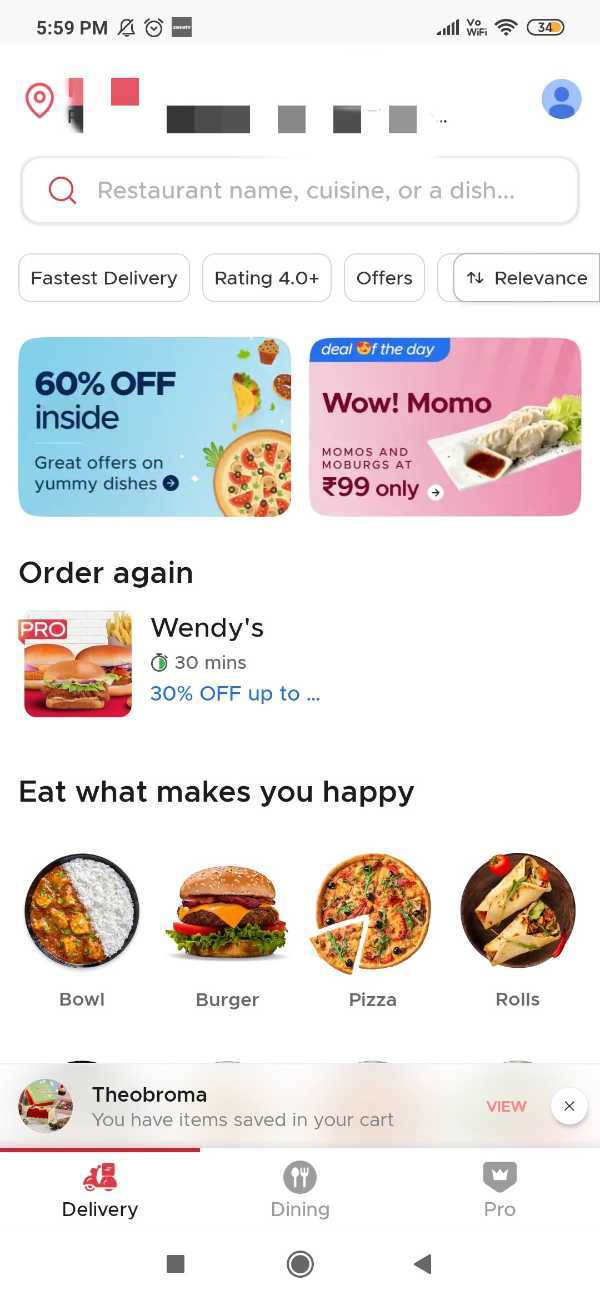This screenshot depicts a user interface of a mobile food delivery service application, although the specific service is not identifiable. The screenshot captures a moment at 5:59 p.m., as indicated by the time display in the top left corner. Adjacent to the time, there are various notifications icons: an indication that notification sounds are off, a timer application, and another undetermined app notification. On the right side of the status bar, icons for data strength, VoWiFi, WiFi connectivity, and battery life at 37% are visible.

The main screen of the app features several elements. At the top, there is a search bar that invites the user to input restaurant names, cuisines, or dishes. To the top right of the search bar, a profile picture icon suggests user personalization or login actions.

Underneath the search bar, the app provides filter options such as "Fastest Delivery," "Rating 4.0+," and "Offers," alongside a button to sort search results by relevance. Following this, there are two promotional banners. One banner offers "60% off" and promotes restaurants like "Wow Momo" and a special for "Moberg's at 99." Images included show diverse food items including a pizza and some dumplings.

The section below is labeled "Order Again," with Wendy's being highlighted as a repeat order suggestion. Further down, there is a motivational prompt saying, "Eat what makes you happy," followed by a visual menu displaying various food categories such as bowls, burgers, pizzas, and rolls.

At the bottom of the screen, there is a notification from the app’s interface: "Theo Roma, you have items saved in your cart." Below this message, three navigation options are provided to the user: "Delivery," "Dining," and "Pro."